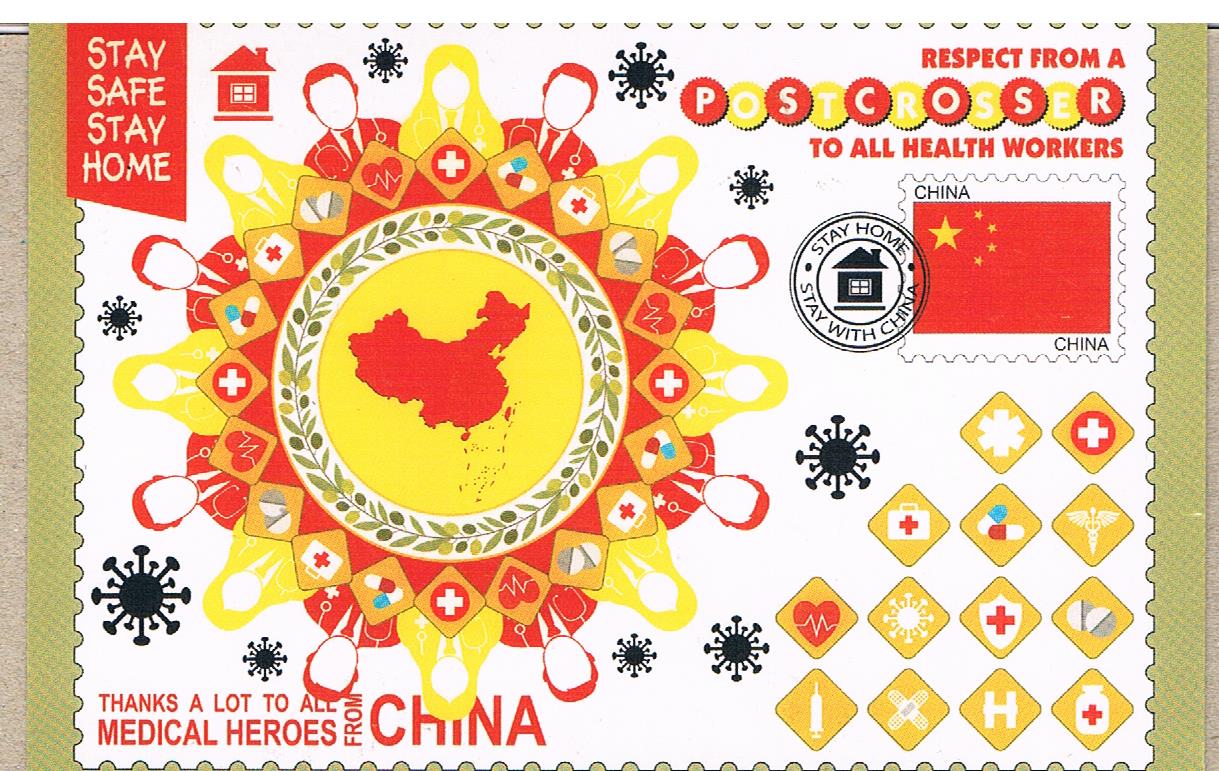This detailed postcard, crafted in vivid colors, primarily white with accents of red, yellow, and black, embodies a heartfelt tribute to healthcare workers, particularly those from China. At the top left corner, it prominently displays the message "Stay Safe, Stay Home" in striking red text accompanied by a small house illustration. Adjacent to this, "Respect from a Post Crosser to All Health Workers" is highlighted, with each letter of "post crosser" set against alternating red and yellow backgrounds. Central to the design is a drawn map of China encircled by representations of healthcare professionals—men in red attire with stethoscopes and badges, and women in yellow. Surrounding them are delicate illustrations of stars or snowflakes. Below, the sentiment "Thanks a lot to all the medical heroes from China" is expressed. Flanked by medical symbols such as a heart, first-aid kit, band-aids, syringe, shield, and Red Cross, this symbolic imagery emphasizes the theme of healthcare. At the bottom, the postcard also features the Chinese flag with the words "Stay Home, Stay with China," underscored by a motif of laurel wreaths, enhancing the sense of appreciation and solidarity.